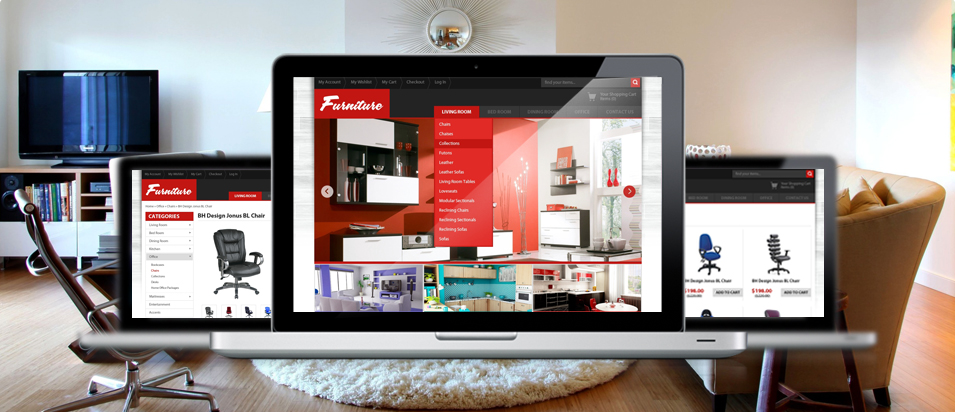The image depicts a beautifully decorated modern home with a relaxed atmosphere. On the right-hand side of the living room, a television is positioned on a shelving unit stocked with books. A comfortable, relaxed computer chair suggests a space designed for both leisure and productivity. The living area features a white, fuzzy circular rug that adds a cozy touch, while a tan leather couch sits invitingly on the left-hand side. Behind the couch, either a clock or a decorative mirror with a sunburst design adorns the white walls, adding an artistic flair to the room. The hardwood floor enhances the room's warm and inviting ambiance. Although partially obscured, there appears to be a poster on the left-hand side, adding a personalized touch to the décor.

Prominently featured in the foreground are three computer screens, displaying furniture options available for purchase on a website. The first and third screens, both smaller in size compared to the middle one, showcase images of armchairs and desk chairs on rolling bases. The larger, central screen shares the same furniture logo and drop-down menu as the others but offers a more comprehensive view, showing different rooms of a house. The rooms displayed include a kitchen, a living room, an office space, and specifically highlight an office setup. This central screen serves as the focal point, blending seamlessly with the room's contemporary aesthetic while providing a glimpse into stylish home furniture options.